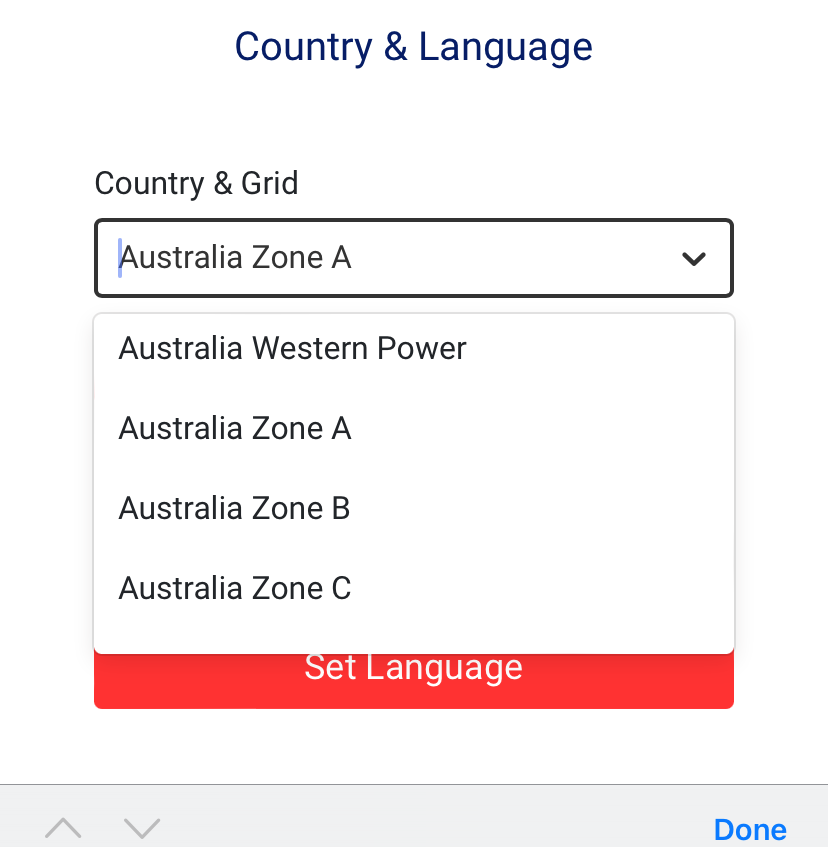Website Interface Preview:

The image showcases a website interface related to selecting a country and language, featuring a simple and compact layout. The top section, set against a clean white background, displays blue text that reads "Country and Language." Directly below, in black text, it states "Country and Grid," followed by a drop-down menu with the option "Australia Zone A" selected. 

Continuing below, the interface lists several options, all in black text:
- "Australia Western Power"
- "Australia Zone A"
- "Australia Zone B"
- "Australia Zone C"

Beneath these options, a red bar with white text prominently displays the button "Set Language." 

The bottom section of the image is a gray bar containing two arrows—an up arrow and a down arrow—allowing users to scroll through the options. In the lower right-hand corner of this gray strip, the word "Done" appears in bright blue letters, indicating the completion of the selection process.

This compact image effectively presents a straightforward country and language selection interface, with all necessary controls and options clearly laid out.